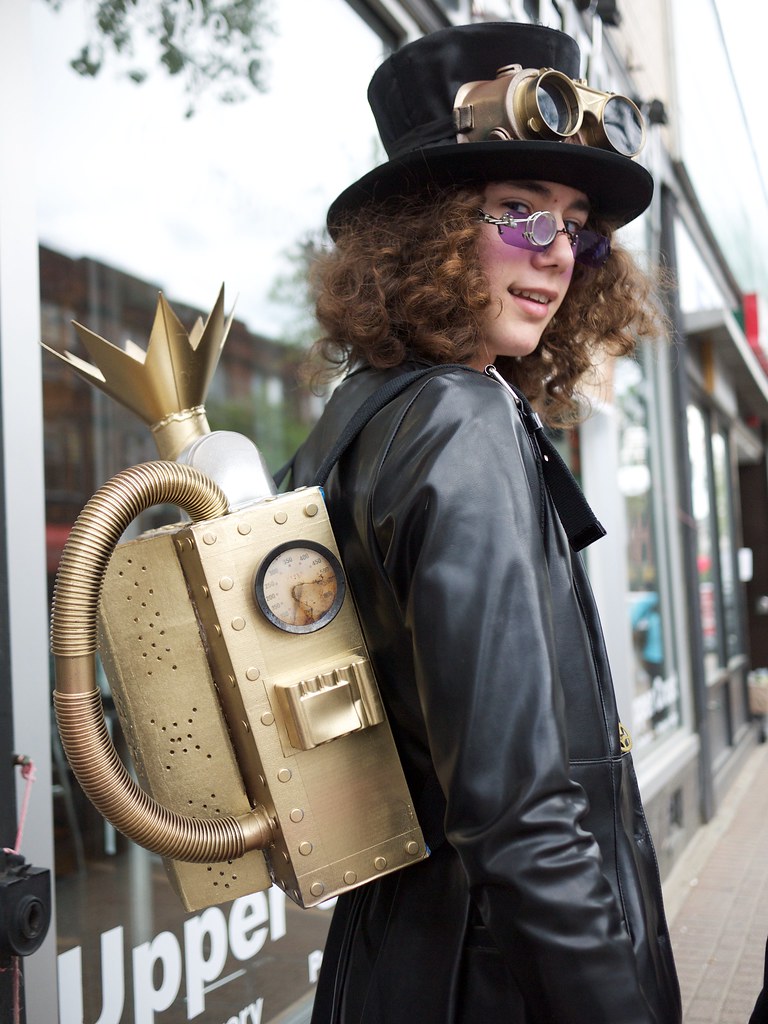The photo captures a young man with a lighter skin complexion and curly red hair, dressed in an elaborate steampunk costume, standing in front of a retail space during the daytime. He sports a black top hat adorned with metal binoculars or glasses with gold lenses, and a purple steampunk visor attached to the hat. His ensemble includes a black long-sleeved leather jacket, and he carries a distinctive steampunk backpack made of gold metal, complete with a pressure gauge on the side. The well-lit, colorful image highlights the glass storefront in the background, providing a clear and vivid view of his detailed costume and the surrounding environment.